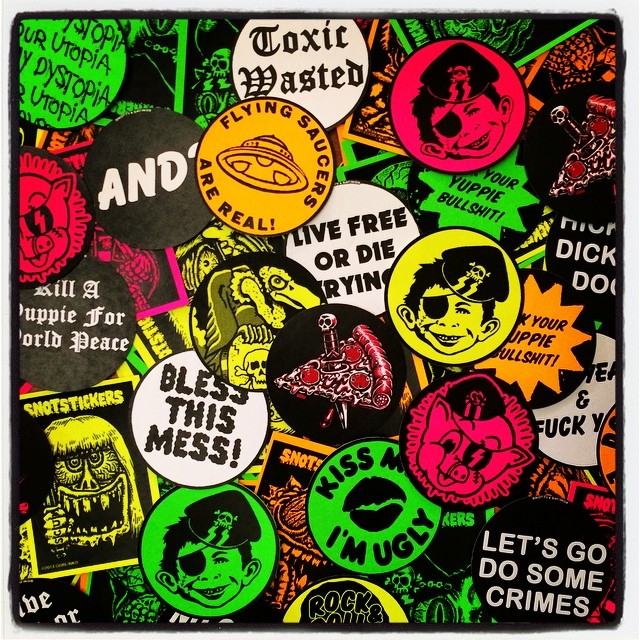The image resembles a vibrant and eclectic CD cover, presenting a chaotic yet intriguing collage of predominantly circular pins and stickers, each with unique and colorful designs that range from bright oranges, yellows, and greens to stark blacks. Central themes include humor, rebellion, and pop culture references. Notable pins include the iconic Mad Magazine boy sporting a pirate eyepatch and cap, a provocative pin that reads "Bless This Mess," and another that asserts "Flying Saucers Are Real," featuring a flying saucer illustration. There is also a pin displaying a slice of pepperoni pizza skewered by a dagger with a skull on the handle, and slogans like "Toxic Wasted" and "Live Free or Die Trying." Additional pins feature quirky messages such as "Kiss Me, I'm Ugly" and "Let's Go Do Some Crimes," topped off with a peculiar "Kill a Puppy for World Peace" button. These various pins overlap in a seemingly haphazard manner within the square frame, creating a bright and eye-catching depiction, evocative of a collection designed to stand out, possibly under a blacklight given their striking hues and rebellious motifs.